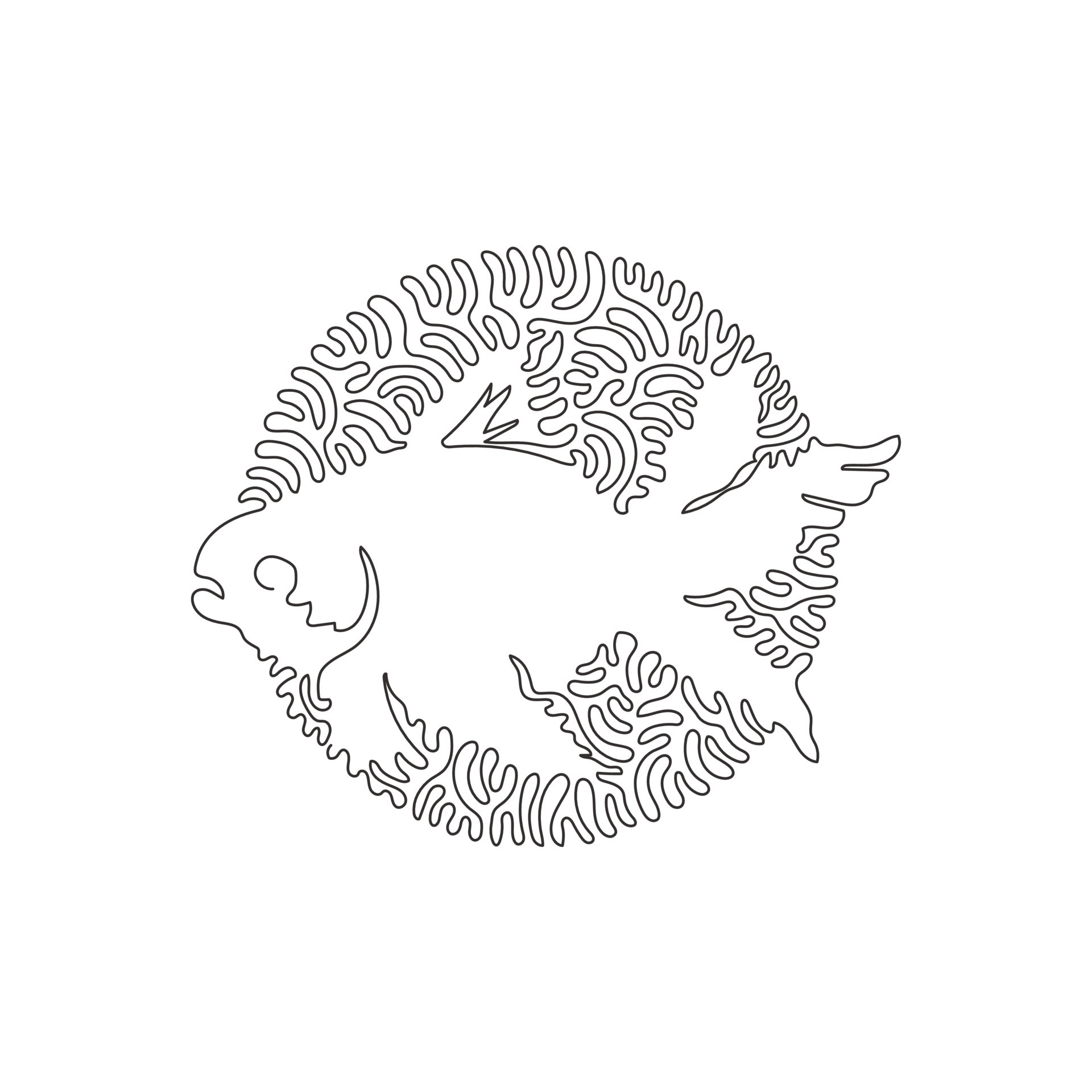This image is a highly stylized drawing of a goldfish in profile, facing to the left with its mouth slightly open. The fish's intricate details include a visible top fin, two fins underneath the front, three fins towards the back, and a prominently protruding tail. The goldfish is embedded within a circular band composed of a tangle of lines, resembling seaweed or coral reef elements, that collectively form the boundary of the circle while partially extending beyond it. The drawing's background is stark white, creating a distinct contrast with the black-outlined fish and seaweed/coral components. At a distance, the goldfish is clearly discernible, but upon closer inspection, it becomes camouflaged within the detailed and connected lines of the surrounding circle. The image does not contain any text.